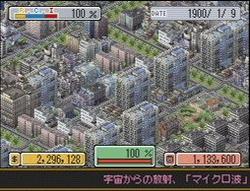The image appears to be a small, grainy, low-resolution depiction, possibly from a smartwatch or a digital illustration. It displays a detailed map of a city area spanning several blocks or up to half a square mile. A prominent broad boulevard runs diagonally from the top left to the bottom right, flanked by either a park or skyscrapers, giving the impression of a green and urban blend. The scene includes other green spots scattered throughout, hinting at parks or public spaces. 

In the top left corner, there’s some text indicating "100%", which might suggest a game statistic. The top right corner displays "date" followed by "1900/1/9," potentially indicating a time of 7:00 PM and a date of January 9th. The bottom left corner features a dollar sign next to a yellow rectangle labeled "2296128", likely representing a game currency or score. Alongside it is a green rectangle with a red stripe marked "100%", and a pink rectangle stating "1", suggesting different statuses or player indicators.

The bottom portion of the image contains a black bar with pink Japanese text, part of which might read "micro..." and possibly "gakko" (meaning school in Japanese). This setup hints at a sim-type game, possibly a real estate simulation game, with different in-game elements and player indicators displayed on the screen.